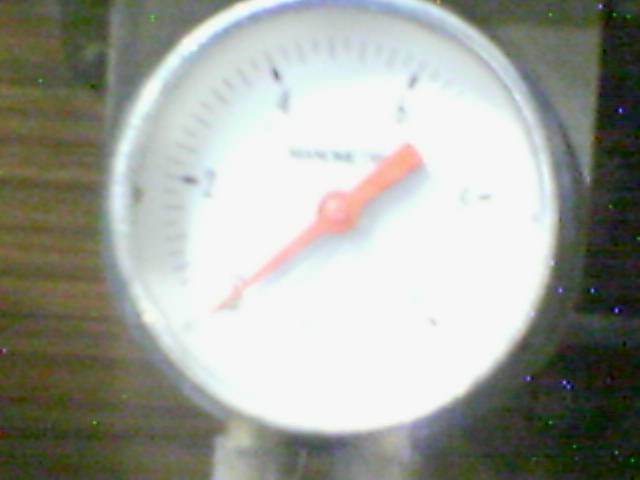This image features a close-up view of a produce scale, typically used for weighing food items such as meat or vegetables. Despite the blurriness, certain details are discernible. The scale has a white face encircled by a silver rim. A red needle, which indicates the weight, spans a range from one to about five pounds, with the number four faintly visible while the number five is obscured. The scale appears substantial in thickness and features two extensions descending from its base. The back of the scale is silver. Its positioning is unclear, as it could either be standing on a surface or hanging; however, it is situated on a wooden surface with visible horizontal lines, suggesting it might be placed on a wooden floor. The side of the scale also shows a black area. The needle is at zero, indicating that no items are currently being weighed.